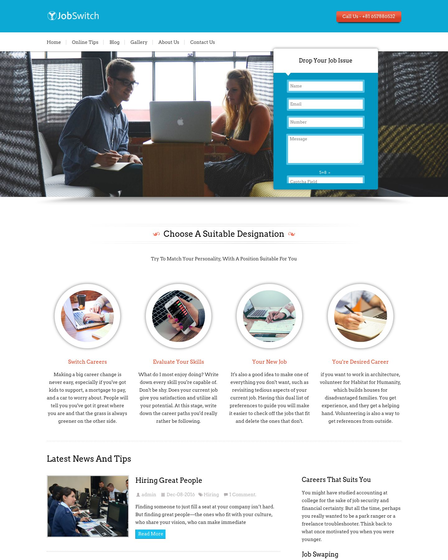The image appears to be a screenshot from the website Jobswitch. The top features a blue border with the word "Jobswitch" written in white in the left corner. On the far right of the blue border is an orange button, possibly labeled "Call Us."

Beneath the blue border is a photograph of a man and woman looking at a laptop together. Above this image is a navigation menu with the options: Home, Online Tips, Blog, Gallery, About Us, and Contact Us.

To the right of the woman in the photo, there is a form area with the heading "Drop Your Job Issue." The form includes fields for Name, Email, Number, and a Message box.

Below this section is a white area titled "Choose a Suitable Destination," featuring four circles, each with an image and a description beneath them. The images depict various job-related activities: one shows a computer, another a person holding a phone, and the last two show people taking notes. The descriptions under the images read: Switch Careers, Evaluate Your Skills, Your New Job, and Your Desired Career, respectively.

At the bottom of the image is a section labeled "Latest News and Tips."